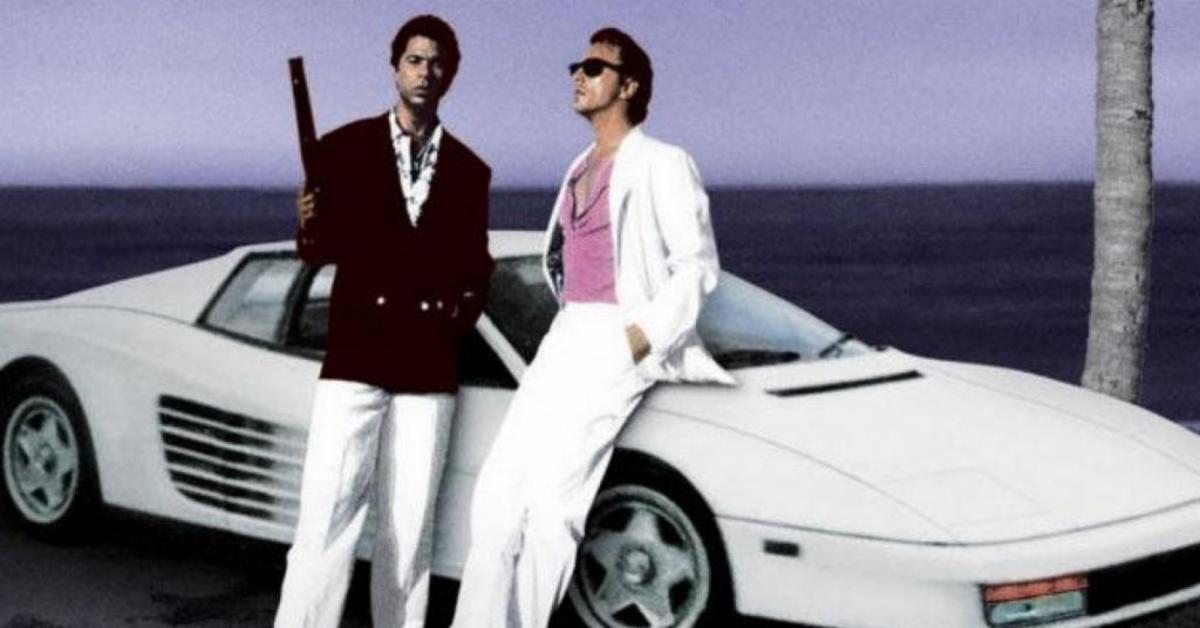The image is an older, grainy photograph set outdoors during the evening, capturing a distinctly vintage 70s vibe. It features two actors, likely from the TV show "Miami Vice." The scene is set against a backdrop of a dark green field under a purple sky, with the ocean visible in the distance and a gray tree trunk on the right.

In the center of the image stands a black man with short black hair, dressed in a black jacket and white shirt. He holds a large rifle in his right hand and looks directly at the camera. To his right is Don Johnson, a white man wearing black sunglasses, a white jacket, and white pants, with a purple t-shirt underneath. His hands are casually tucked into his pockets as he leans against a two-door white sports car, possibly a Ferrari or Lamborghini. Don Johnson is looking slightly upwards and to the side, adding to the cool, composed aura of the scene.